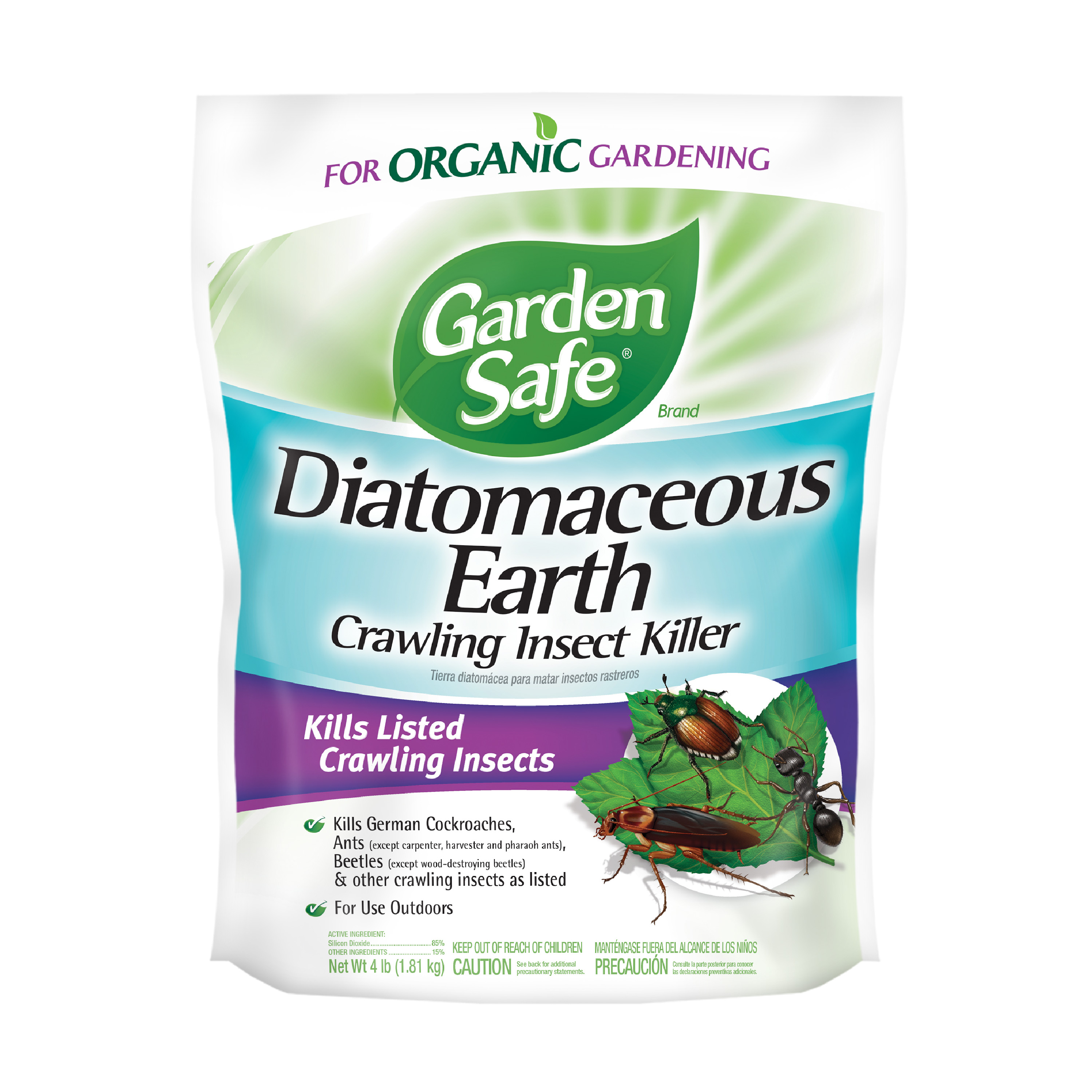This image features the packaging of a "Garden Safe" brand Crawling Insect Killer made from diatomaceous earth. The bag is set against a white background. At the very top of the bag, "For Organic Gardening" is prominently displayed on a white strip, with the word "Organic" in larger, green text. Below this, a green, stylized leaf showcases the brand name "Garden Safe" in white letters. The central part of the bag features a blue section with "Diatomaceous Earth Crawling Insect Killer" in large letters, emphasizing the product name. Beneath this is a purple banner stating "Kills Listed Crawling Insects," accompanied by an illustration of a green leaf with three large bugs: a cockroach, a large ant, and a beetle. Further down, more text explains that the product "Kills German Cockroaches, Ants, Beetles, and Other Crawling Insects as Listed for Use Outdoors." The bottom of the bag contains smaller text including caution labels, weight information, and various warnings, all printed on a white background.